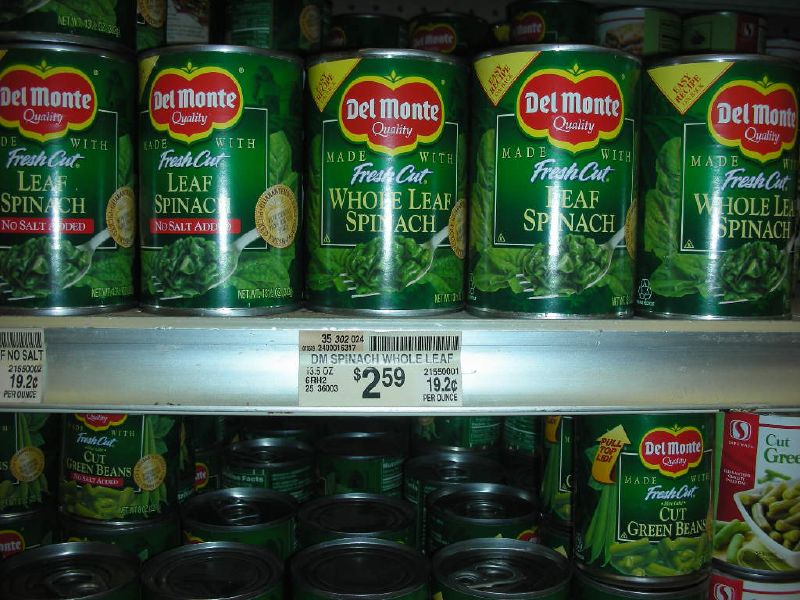The image is a detailed photograph of a supermarket shelf displaying Del Monte products. The shelf features a metallic silver front with a clear white label containing black text that provides the product description, price, and price per ounce, along with a barcode on the top right corner. Showcased prominently are green cans of Del Monte Fresh Cut Whole Leaf Spinach with no salt added, identifiable by their green labels and distinctive red Del Monte logo with a yellow border. Each can, featuring a silver top and an image of spinach on a fork, has a tagline that states "Made with fresh cut whole leaf spinach." Below this row, there is another shelf displaying more Del Monte products, specifically Fresh Cut Green Beans. The price tag on the spinach cans indicates they are priced at $2.59 each and 19.2 cents per ounce, with a specific note for no salt added. The organized and clearly labeled display highlights Del Monte's commitment to quality and transparency in their product offerings.